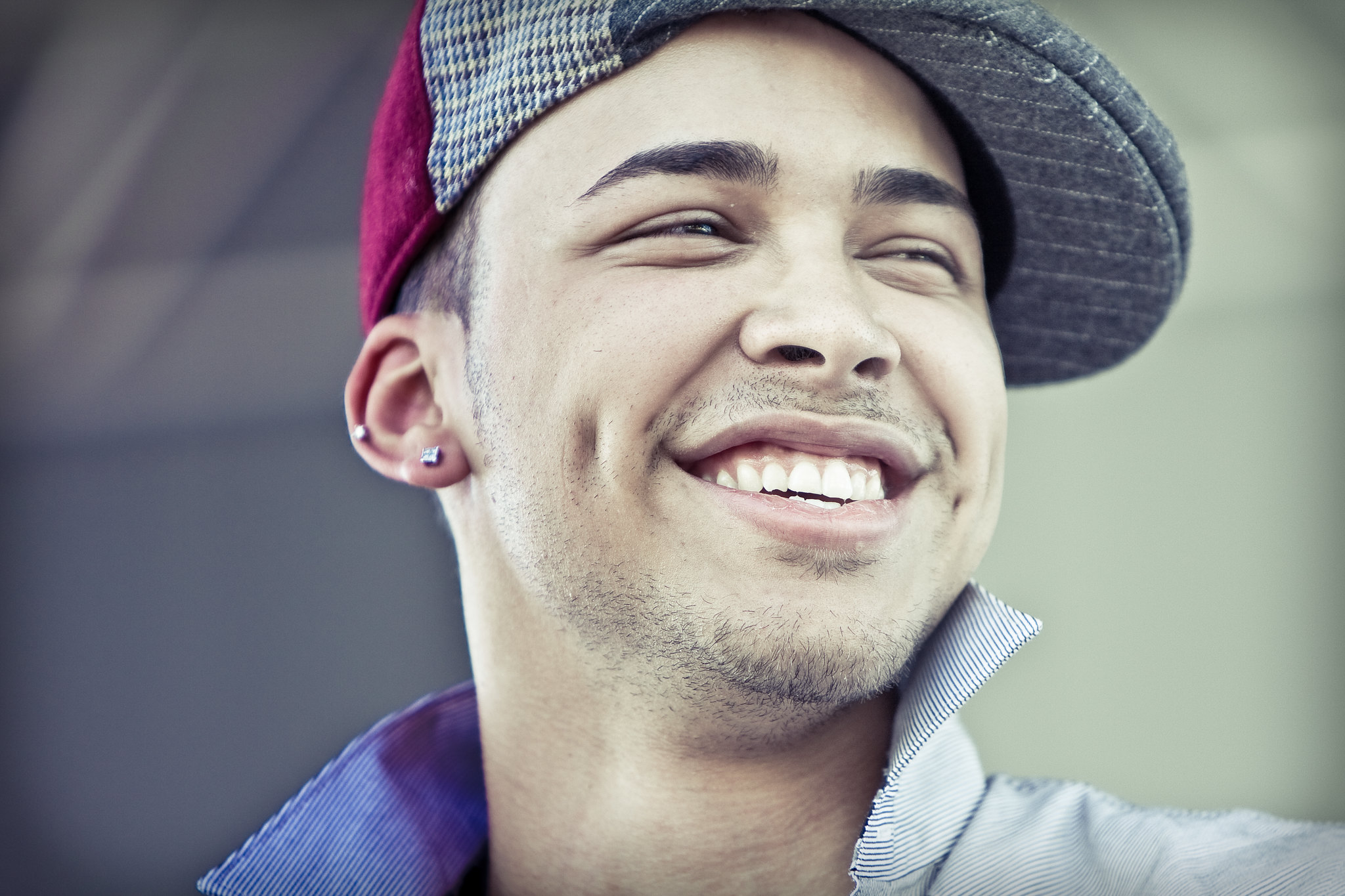This photograph features a young man, likely between 18 and 20 years old, beaming a broad smile that reveals his straight, white teeth. He is wearing a distinctive ball cap made of various patch-colored wool fabrics, with a notably smaller bill and a burgundy-colored back. The hat is slightly off-centered to the right on his head. His right ear, the only one visible, sports two earrings: one in the earlobe and one higher up on the ear's curve. He has dark, short hair, dark eyebrows, and dark eyelashes, along with a modest one or two-day stubble covering his jaw and mustache area. The young man is dressed in a white button-up shirt with tiny blue stripes, and his collar is turned up, revealing the blue striped inner fabric. The background of the image is muted with a blend of gray, lime green, and olive hues, creating a soft, indistinct palette. The overall image has a slightly wider-than-tall dimension, suggesting a relaxed and casual portrait setting.